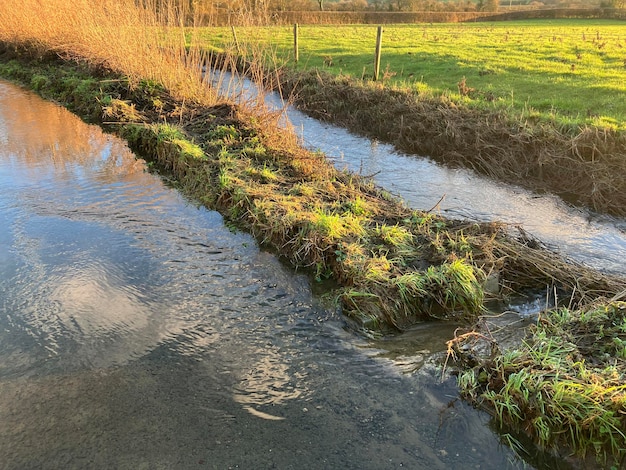The painting depicts a picturesque natural landscape centered around a unique waterway. Dominating the scene is a river stretching across the canvas, with waters varying in hues from deep blue to gray, reflecting the surrounding scenery. To the left of the main river is a narrow, parallel water trench, separated by a thin strip of land adorned with overgrown green vegetation and patches of tall, brownish-yellow grass. Nestled on this slender median, the lush greenery contrasts with the vibrant, golden weeds that exceed the viewer's line of sight at the upper edge. On the right bank of the trench, wooden fence posts stand in a bright green field that extends into a leveled expanse. In the distance, a slight backdrop of a forest adds depth to the landscape, enhancing the scene's serene and idyllic atmosphere.